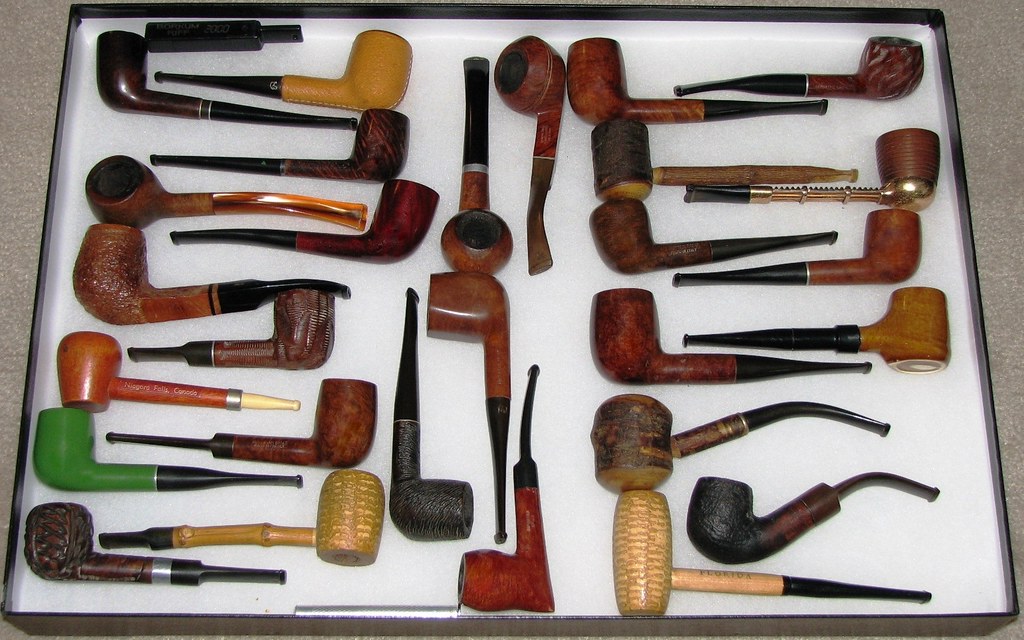This is a rectangular photograph showcasing a meticulously organized collection of antique-style smoking pipes laid out in a tray. The tray, which has a black border and a white bottom—possibly lined with paper or wax paper—rests on a gray surface, perhaps a countertop or desk. The pipes are arranged in a visually striking manner, with distinct sections: on the left, the pipes are arranged horizontally; in the center, they are oriented vertically; and on the right, they are again laid out horizontally.

The collection includes a variety of pipe styles, each with unique characteristics. The stems, where one would place their mouth, are primarily black plastic, but there are also sections with tortoise shell-colored, beige, and metallic stems. The bowls of the pipes, where tobacco is placed and lit, are made from different materials such as carved wood, corncob, and even metal. Among these, there is a noticeable green pipe positioned on the left side.

Noteworthy among the collection are bent and traditional straight pipes—some reminiscent of those used by Sherlock Holmes—and pieces that appear to be made from briar wood. At least twenty-five pipes are displayed, making this a comprehensive and varied collection likely intended for display.